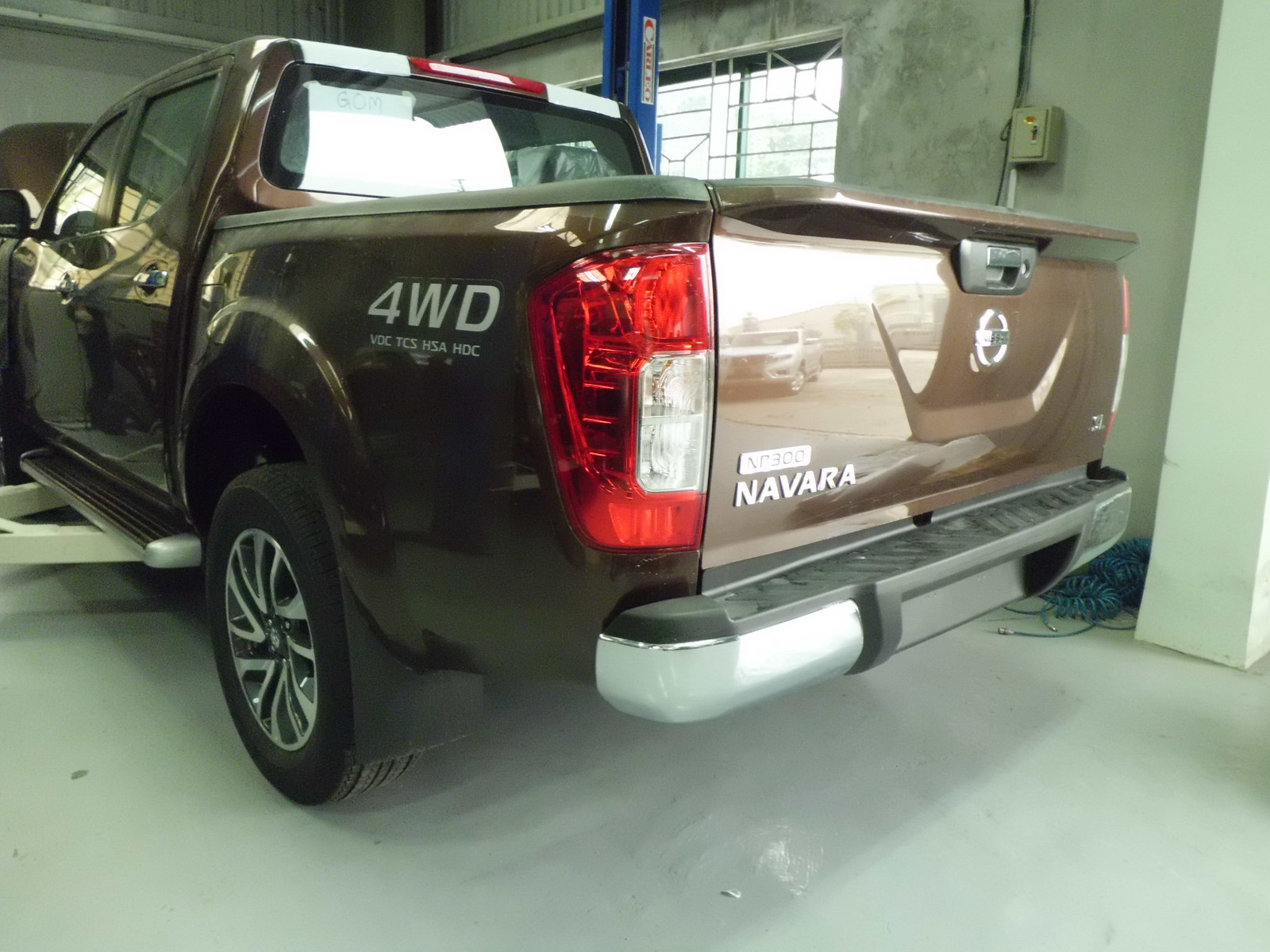This photograph depicts a meticulously maintained professional garage, potentially part of a dealership or mechanic shop. The spacious, well-lit garage features pristine white walls and a well-maintained concrete floor. Central to the image is a brand new, coffee-colored metallic Nissan Navara pickup truck, equipped with advanced features like VDC, TCS, HSA, and HDC, positioned on a white metal platform lift. The lift's arm is securely placed under the truck’s underbelly, suggesting it is being prepared for maintenance or inspection. To the right of the vehicle, a blue scaffolding and coiled blue air hoses are visible, hinting at the presence of various tools and equipment typical of a professional repair setting. The overall impression is one of a clean, organized, and expertly run facility.